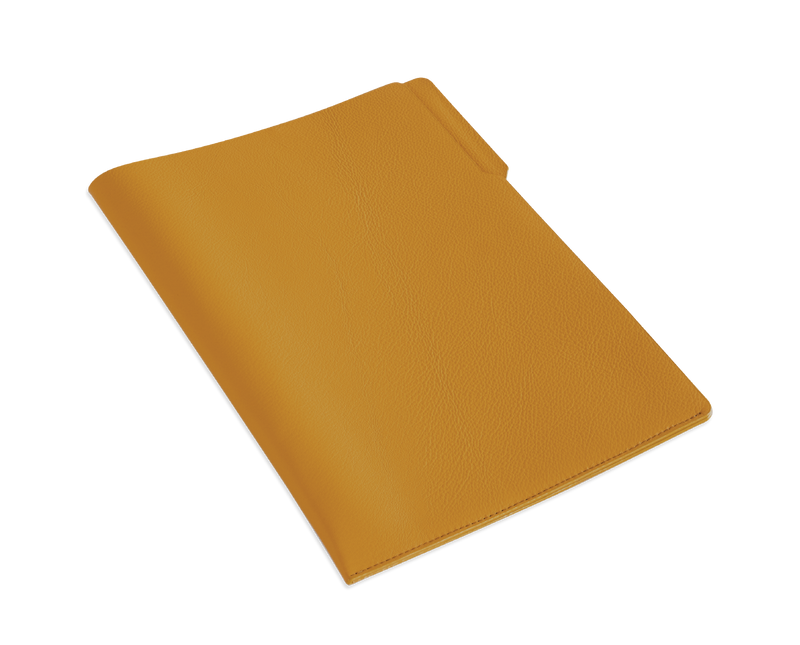This image depicts a textured, medium-brown folder case set against a completely white background. The folder features a tab on the top right corner for labeling purposes, deviating from the usual light beige color of typical manila folders. The material appears to be leather or faux leather, characterized by many small bumps providing a grainy texture. The folder is stitched shut along the bottom edge and has a noticeable crease near the left side, creating a shadow. The top and right sides of the folder remain open, suggesting it functions as a sophisticated sleeve for documents, an iPad, or a smaller notebook.